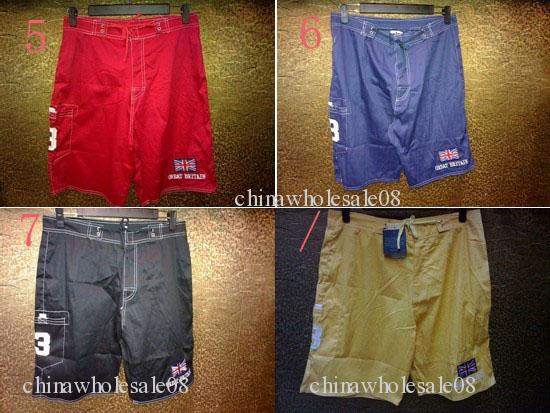The image displays four distinct pairs of men's shorts, each positioned within a separate quadrant of the photograph, forming a rectangular collage. Starting from the top left and moving clockwise, the first pair is red with a Union Jack emblem on the lower right leg and a large number 5 on the upper left of the photograph. The second pair, situated in the top right, is blue and also features the Union Jack on its lower right leg; both the red and blue shorts have noticeable white stitching and the red shorts include a drawstring. Positioned in the bottom right, the beige shorts also showcase the Union Jack on the lower right leg and include a drawstring, set against a notably darker background compared to the others. Finally, the bottom left quadrant houses a black pair of shorts with white stitching and a number 3 next to a faux pocket on the lower left leg, along with the Union Jack lower on the right leg; these shorts are labeled with the number 7. Throughout the image, the watermark "China Wholesale 08" appears three times, once in the center, again on the lower left, and finally on the lower right of the photograph. The varying backgrounds include bronze-like textures and a darker texture for the beige shorts, adding contrast and depth to the presentation.